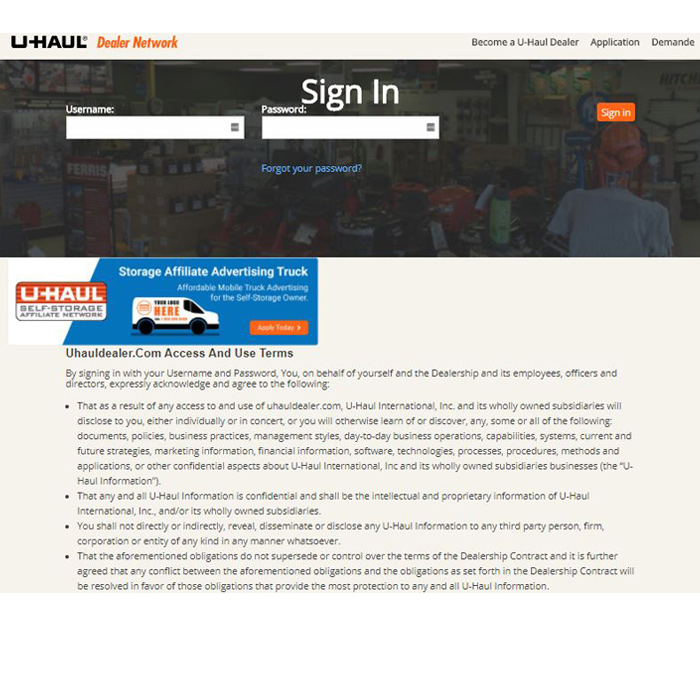The image features a light blue background with the headline "U-Haul Dealer Network" prominently displayed in red. Below the headline, text reads "Become a U-Haul Dealer - Application and Demand." A dark section houses a large input box labeled "Username" and another for "Password," both with white text. Beneath these boxes, there is a red "Sign In" button, and below it, blue text reads "Forgot Your Password?" The image within this dark background depicts various individuals. Moving back to the light blue background, there is a smaller box for the "U-Haul Self Storage Affiliate Network," where "U-Haul" is written in orange with white text, and the bottom part is blue.

A larger blue box follows, proclaiming "Storage Affiliate Advertising Truck: Affordable Mobile Truck Advertising for Self Storage Owners." This section includes an illustration of a white truck decorated in orange and blue hues. An orange button labeled "Apply Today" is displayed prominently. Finally, towards the bottom, in smaller text, "U-HaulDealer.com Access and Use Terms" is noted, followed by a list formatted with dotted lines.